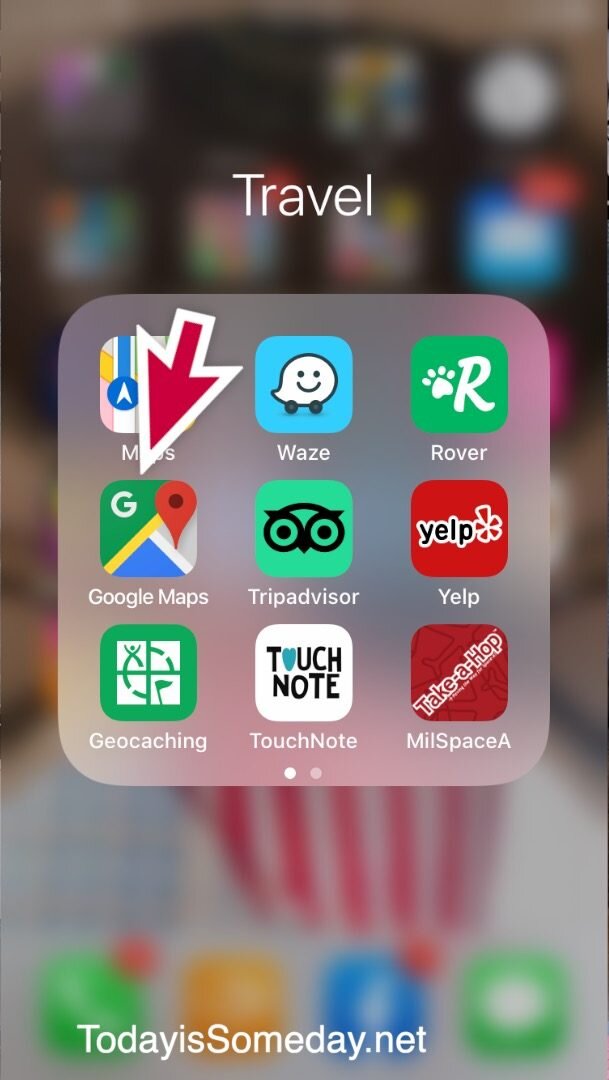In the image, a cell phone's screen is displayed with a blurred background, showing a vague outline of a phone with apps. The top part of the screen is devoid of any status information like time or notifications. Centered about an inch from the top is the word "Travel," prominently displayed in white, with the "T" capitalized.

Below this title, there are three rows of apps, neatly arranged in a 3x3 grid format:

**First Row (Left to Right):**
1. **Maps** - Featuring the recognizable icon with a red arrow.
2. **Waze** - This app has an icon resembling a speech bubble on wheels, with a smiling face.
3. **Rover** - Displaying a green background with a white paw print representing a dog.

**Second Row:**
1. **Google Maps** - The familiar map icon with a simplified pointer.
2. **TripAdvisor** - Represented by an owl’s eyes and beak in black outline on a green background.
3. **Yelp** - Iconized with its traditional bright red background.

**Third Row:**
1. **Geocaching** - Likely symbolized by a location or navigation-related icon.
2. **TouchNote** - Featuring a white icon, specifics unclear.
3. **Take A Hop** - Presenting the text "Mills Mill Space," not widely known.

At the very bottom, there's an app named **TodayIsSomeDay**, though its specific function or icon is not described.

Overall, the arrangement and selection of apps suggest a travel-themed suite intended for navigation, reviews, and travel planning.